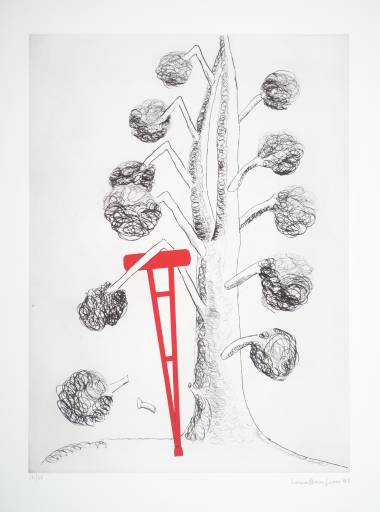This is an unusual and captivating black-and-white ink drawing with a cartoonish feel, depicting a tree with anthropomorphic qualities. The tree, stretching vertically like a traditional tree trunk, is adorned with bifurcating branches on each side, resembling a series of symmetrical legs that arch downward like a creature's limbs. Each branch terminates in a round, lollipop-style head, creating an abstract, almost whimsical appearance. Notably, on the left side of the tree, the second branch from the bottom is bent and propped up by a striking red crutch, adding a pop of color to the otherwise monochromatic scene. The bottommost branch on the left side is broken off, emphasizing the sense of fragility. The backdrop is predominantly white, with subtle gray hues, allowing the intricate black and white swirls of the tree and its "shrubs" to stand out. This composition combines elements of realism and fantasy, drawing attention to its vivid details and unique structure.